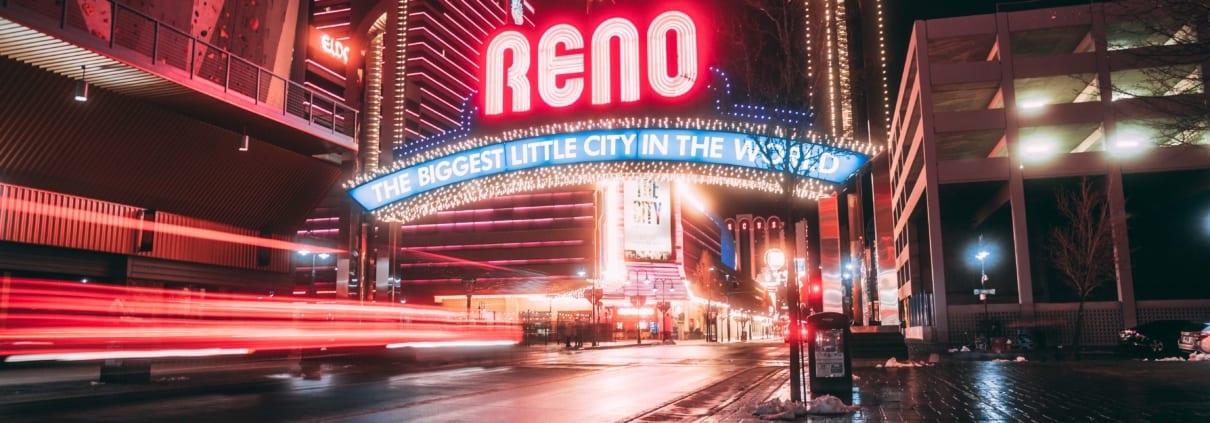This photograph captures a nighttime cityscape of Reno, Nevada, evidenced by the prominent signage. The image, taken in a wide rectangular format, showcases a street devoid of cars, with wet, shiny pavement suggesting recent rain. Dominating the scene is a large illuminated sign stretching across the street, with "Reno" written in large, white bubble letters outlined in red. Directly below this, an arch-shaped sign reads "THE BIGGEST LITTLE CITY IN THE WORLD" in white, all-caps lettering set against a blue background. Both signs are adorned with numerous small, yellow or white lights, reminiscent of Christmas lights.

To the right side of the image, there appears to be a parking garage, characterized by its white lights. The scene is vibrant with illuminated buildings in the background, their lights predominantly pinkish-red or yellowish-orange. On the left, the image shows some streaks and blurred lines of red and yellow, likely indicating a car moving quickly, contributing to a dynamic feel. A building on the upper left features a railing, although the rest of it is blurry.

Although the bright lights make it challenging to see fine details, a few people can be discerned in the distance, dressed in dark clothing. Overall, the street, sidewalks, and buildings contribute to a lively and visually rich representation of Reno at night.